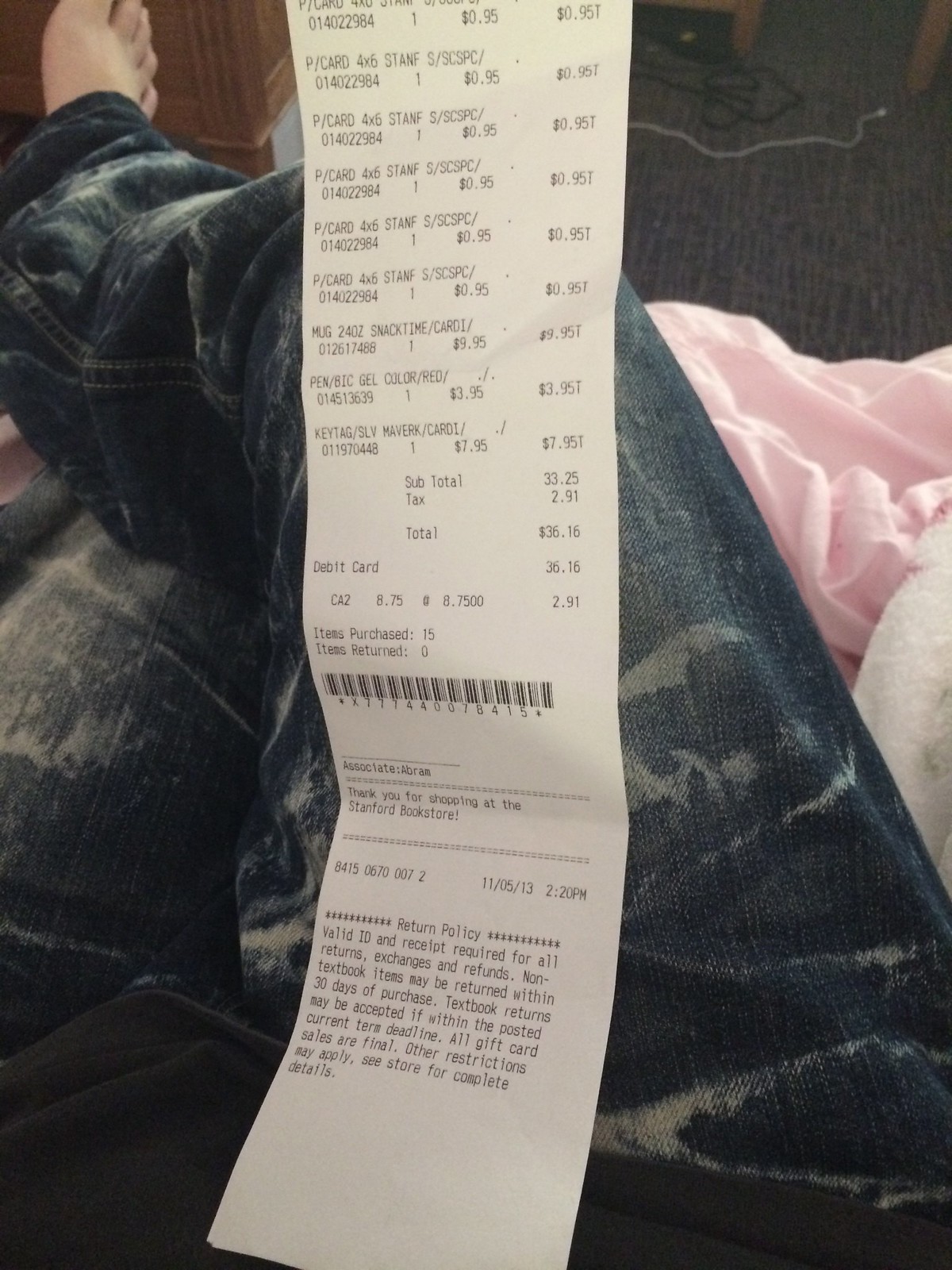In the photograph, a disheveled room with a slightly messy bed featuring a pink crumpled sheet forms the backdrop. The main focal point is a long receipt held up, dangling prominently into the frame from the top. The receipt, with its detailed list of items and prices, cascades over the legs of an individual seated cross-legged, partially obscured by the document. The person is donning overly baggy, acid-wash-style blue jeans adorned with white marks that could either be paint splatters, bleach stains, or part of the design. Their right foot is bare and appears somewhat chubby or swollen. The total of the receipt is $36.16, covering multiple duplicate items priced at $0.95 each, among others ranging up to $9.95. Near the bottom of the receipt, a barcode and extensive return policy text are clearly visible. The room appears to also have laundry strewn about, enhancing the overall sense of casual disorder capturing the everyday moment.